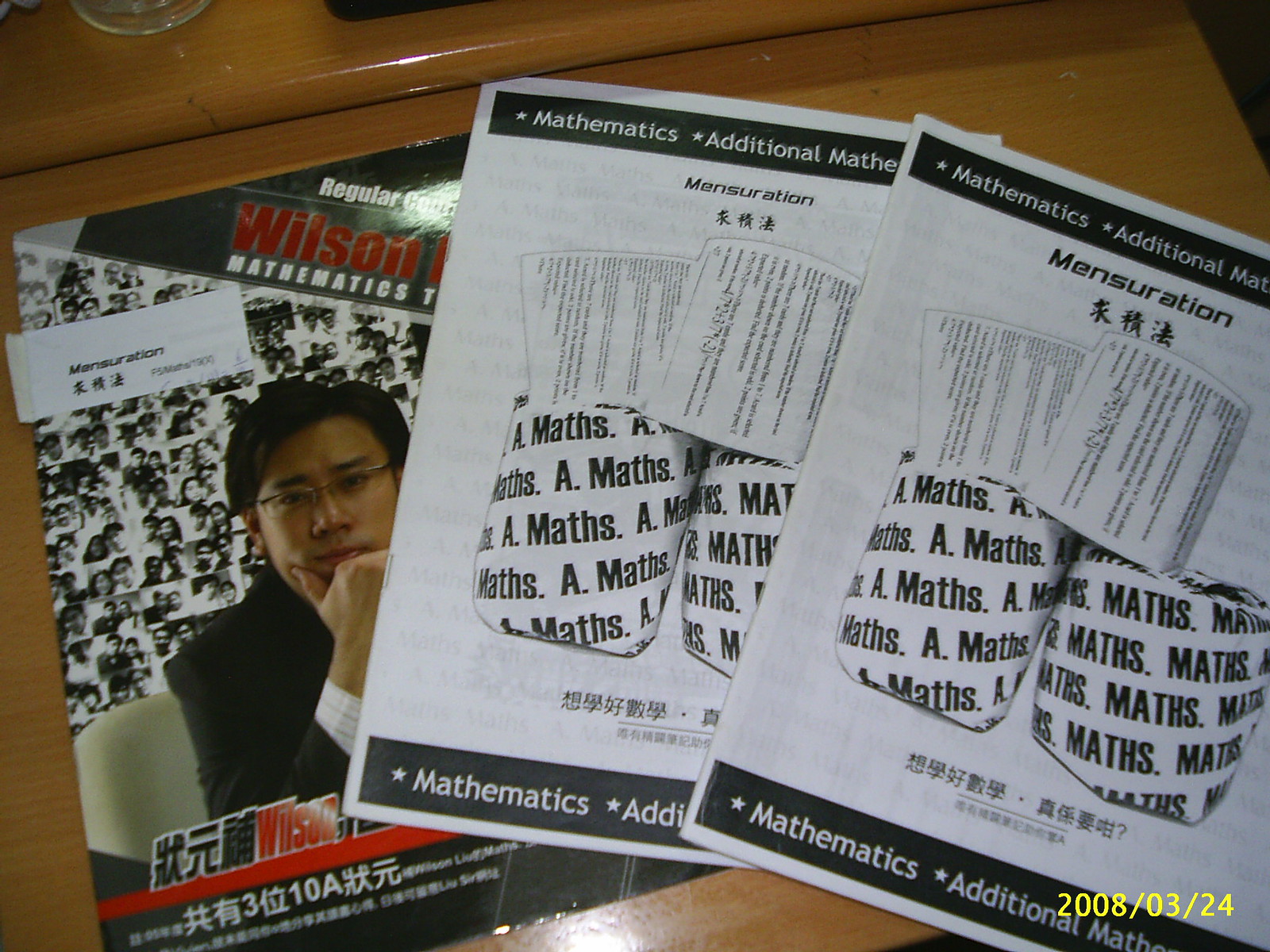In the photograph, a wooden dresser or counter is visible, partially covered by a series of overlapping papers and items. Prominently featured among the papers is a magazine with Chinese writing and an Asian man in glasses and a suit staring directly at the camera. This magazine, which contains several black and white photos, sits beneath two documents titled "Mathematics" and "Additional Mathematics Iteration." Both papers detail mathematical concepts, with legible words including "mathematics" and "mensuration." Additionally, smaller white shapes with writing are partially visible. A yellow timestamp reading "2008/03/24" is marked at the bottom right corner of the image. In the background, there are indistinct items, possibly including a glass, that are only partially in view.